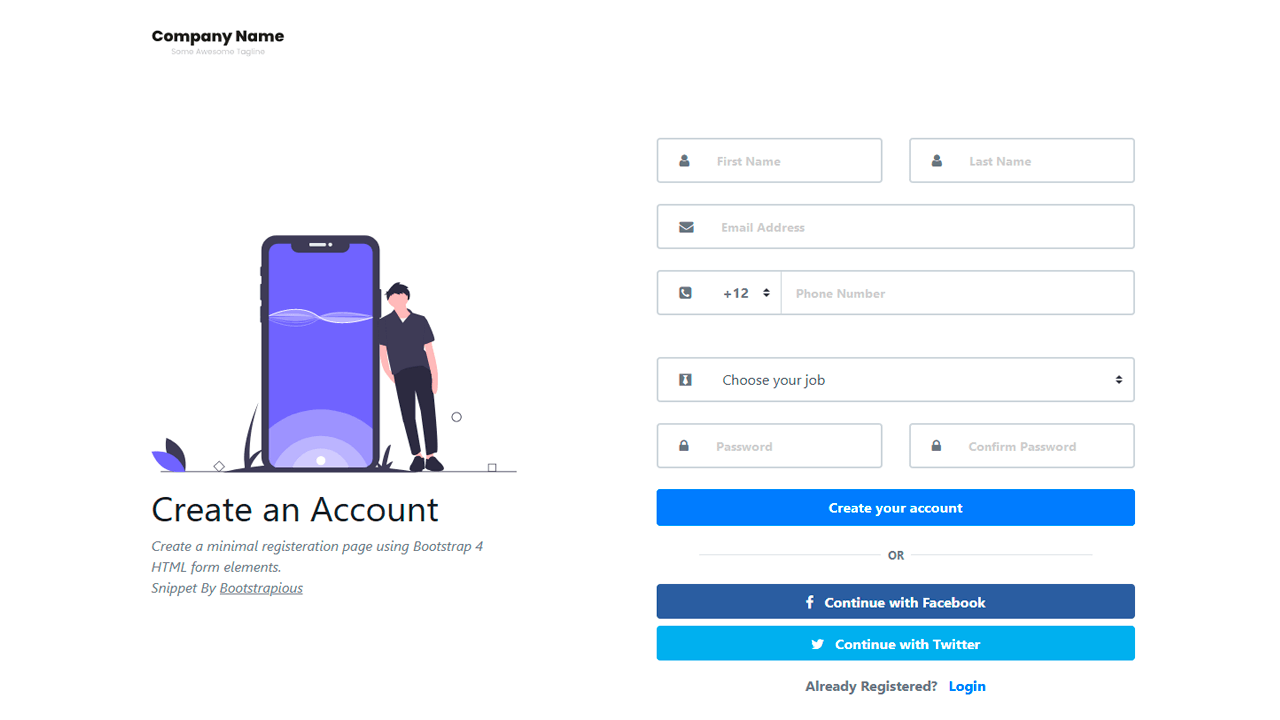Here's a refined and detailed caption for the image:

"On a white background, the company's name is displayed prominently. The foreground features a large smartphone with a vibrant purple screen, against which a man with black hair, dressed in all black, casually leans. The screen of the phone shows a minimalistic registration page designed using Bootstrap 4, HTML form elements, and a snippet by Bootstrap IO. The form fields include placeholders for 'First Name,' 'Last Name,' 'Email,' 'Phone Number,' and a dropdown menu to select a job role. The password field is adorned with a lock icon, and there's a field for confirming the password. At the bottom, users are prompted to 'Create Your Account' via a large blue button or opt to continue registering through Facebook or Twitter. For those already registered, there's a 'Log In' option. The design showcases a palette of white, gray, several shades of blue, purple, and a hint of peach. This pre-made form template can be easily integrated into a website, simplifying the registration process for developers."